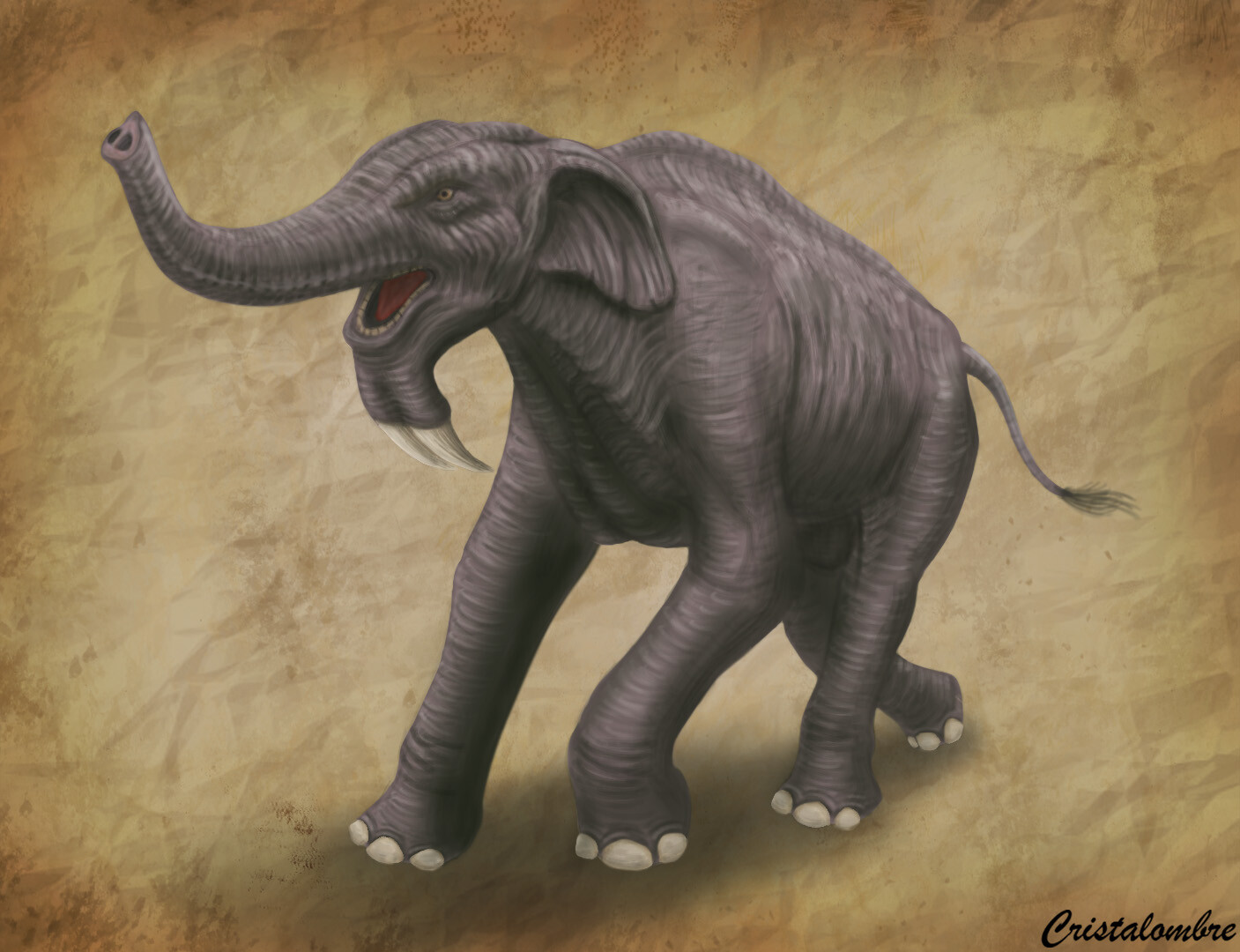The image depicts an elephant-like creature, intricately designed to resemble, but distinctly different from, a traditional elephant. The creature occupies the entire frame, characterized by several unusual features. Notably, it has two large horns protruding from its chin, curving back towards its neck, and an emaciated frame with a highly pronounced spine. The legs are abnormally long for an elephant, and the front legs are particularly elongated. Its skin appears loose and stretched, with misplaced lines and wrinkles that contribute to its eeriness.

The background resembles aged, wrinkled parchment, reminiscent of old, weathered paper, possibly crumpled and dirtied, with darkened edges and splotches. This background enhances the antique and otherworldly feel of the image. In the bottom right corner, the artist's name, Crystal Lombre, is inscribed in a modern cursive style, anchoring the image in contemporary digital artistry despite its archaic aesthetic. Overall, the image strikes a balance between a traditional sketch and a strategically aged, computer-generated creation, blending historical and modern artistic techniques.